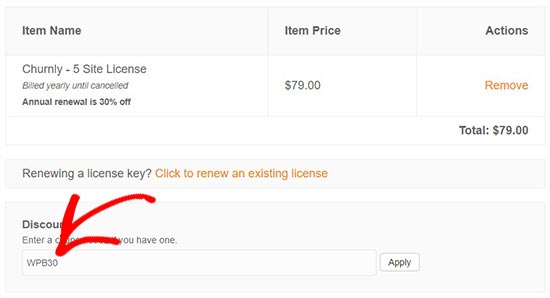This screenshot captures a portion of an online shopping cart page with a white background. At the top, there is an information section showing three columns, each labeled in dark gray text with a light gray header. The columns are labeled "Item Name," "Item Price," and "Actions."

In the first row under these headers, the content is divided by thin gray lines. 

1. Under "Item Name," in medium gray text, it reads "Churnly - 5 Site License," followed by italicized text stating, "Billed yearly until canceled." Below this, bolded in smaller text, it says, "Annual renewal is 30% off."
2. In the "Item Price" column, it lists $79.00.
3. Under "Actions," the text reads "Remove" in noticeable orange.

Beneath this table, a single row displays the total cost on the far right in bolded text: "Total: $79.00."

Below this, a light gray rectangle separated by a small white margin includes text on the left side that reads, "Renewing a license key," with "Click to renew an existing license" in orange on the right.

Further down, another gray rectangle features bolded text "Discount" at the top left. Below this, there is a partially obscured line of text starting with "Enter A" and ending with "you have one," overlaid with a red arrow pointing to a text box beneath. Within the white text box, gray lettering displays "WPB30." To the right of the text box, a light gray box outlined by a thin gray line contains the word "Apply" in gray text.